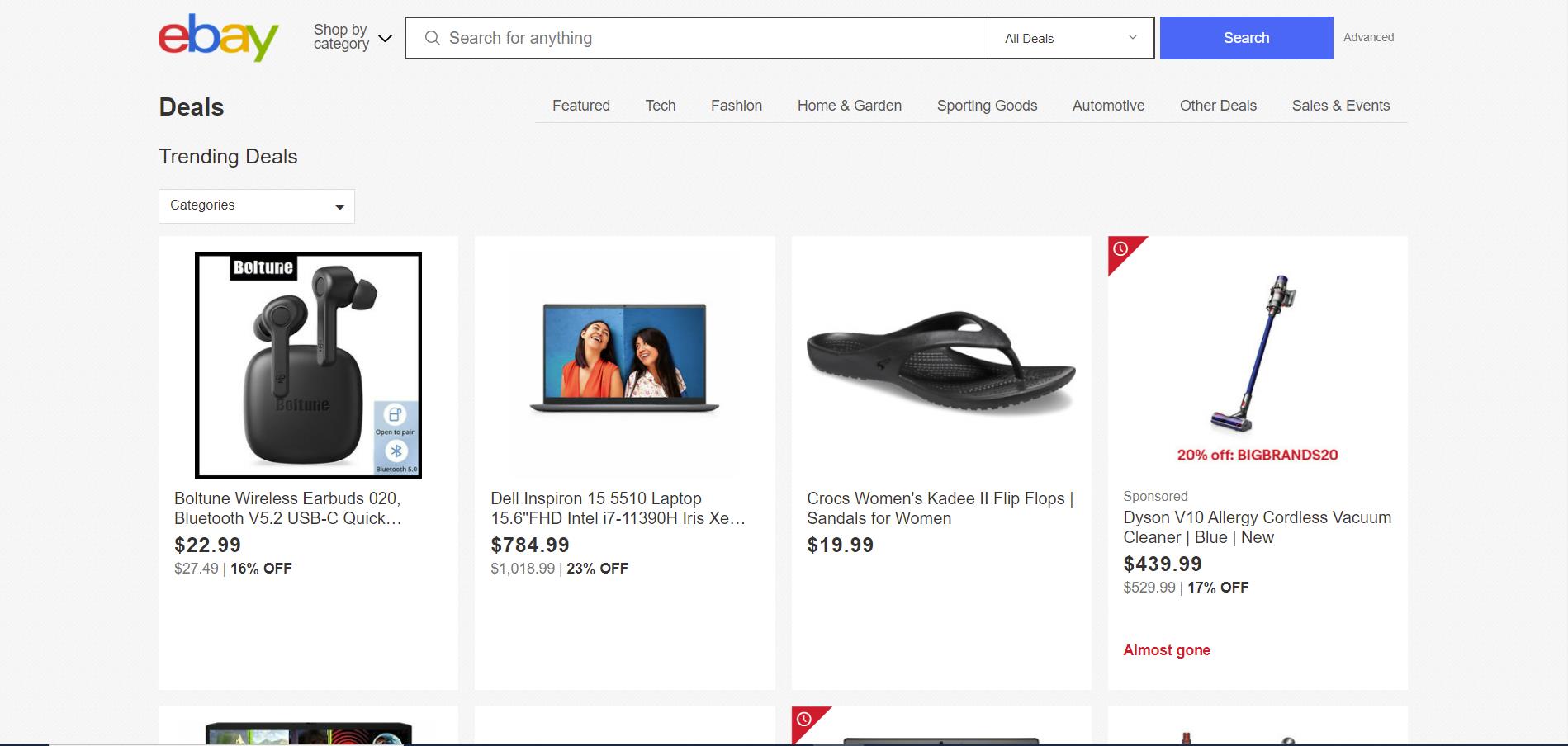This image is a detailed screenshot of the eBay homepage showcasing the various sections and promotional deals available at the time. 

At the top of the page, the eBay logo is prominently displayed alongside navigation options such as "Shop by Category." Next to these options is a search bar with the placeholder text "Search for anything," accompanied by a blue search button. The search bar is currently empty. Below these elements, there are multiple links to different sections, including "Deals," which further break down into categories like "Featured," "Tech," "Fashion," "Home & Garden," "Sporting Goods," "Automotive," "Other Deals," and "Sales & Events."

The "Trending Deals" section features four boxed images highlighting the following items:

1. **Boltune Wireless Earbuds**: These Bluetooth 5.2 earbuds, priced at $22.99 with a 16% discount, are showcased with an all-black design including the carrying case.
2. **Dell Inspiron 155510 Laptop**: Priced at $784.99 with a 23% discount, the image shows a laptop displaying a screen with two smiling people.
3. **Crocs Women's KDU 2 Flip-Flops**: These women's sandals are available for $19.99.
4. **Dyson V10 Allergy Cordless Vacuum Cleaner**: Listed at $439.99 with a 17% discount, this blue vacuum cleaner is also eligible for an additional 20% off using the coupon code "BIGBRANDS20."

Each product’s image is accompanied by its description, price, and percentage discount. The Dyson vacuum’s promotional coupon highlights further savings potential. This well-organized layout assists users in easily navigating deals and categories on the eBay platform.